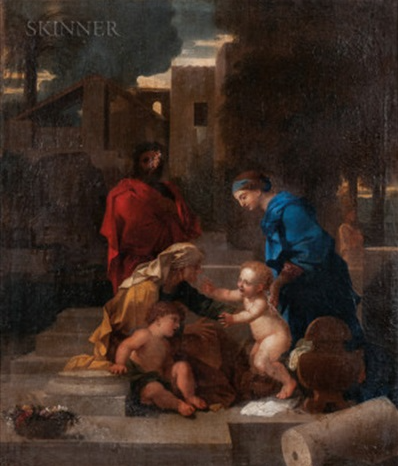The painting appears to be a somber, Renaissance-style piece characterized by its faded and blurry appearance. Vertically aligned and rectangular, the artwork features an inscription at the very top, in all capital letters, reading "SKINNER" in grey. The scene is set against a backdrop of antiquated, brown-hued stone buildings with glimpses of a dusky sky, tinged with pink and grey clouds, suggesting a sunset. The upper right side of the painting is a nebulous blur of brown, hinting at trees.

Centrally, there are five figures. A prominent, large man, possibly Joseph, dressed in a vivid red robe, stands or kneels behind a group. His face is indistinct and deformed-looking. Opposite him is a woman in a stunning blue dress and headband, identified as Elizabeth. She is attentively hunched over, holding a naked baby with curly hair, thought to be John, who reaches out towards her. Next to her, another small boy with minimal clothing sits. Seated among the figures is a figure in a dark yellow garment, likely Mary, who is also looking down at the children. The adults and children appear to be arranged on stone steps, creating a symmetrical composition on what looks like a concrete foundation amidst the older stone setting. The rich, dark shades of grey, brown, and red imbue the painting with a somber, reflective mood.